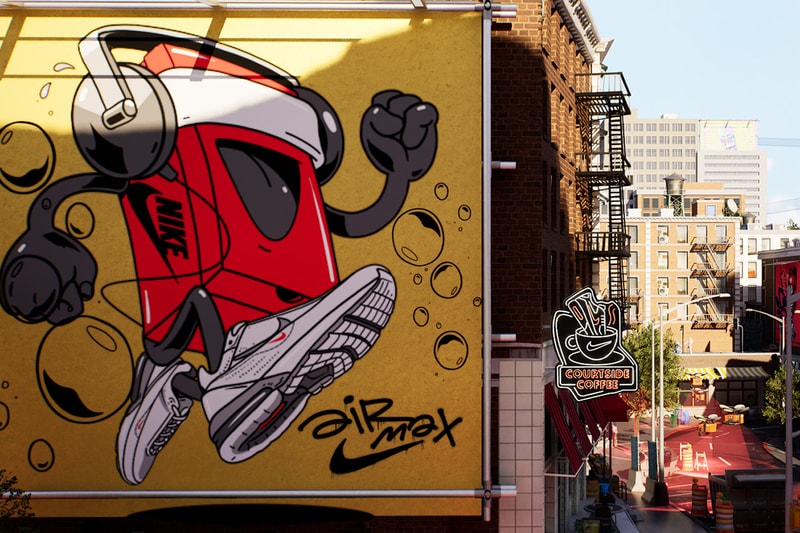The image captures a vibrant urban scene viewed from an elevated vantage point, showcasing a bustling corner of a street dominated by a striking Nike advertisement. The left side of the image features a large, vivid billboard with a yellow background depicting an animated Walkman character adorned with Nike branding, complete with headphones, arms, and legs wearing white and red Nike Air Max sneakers. The character also has a distinctive headband where its eyes would be.

Adjacent to the billboard, to the right, there is a detailed brown building with visually prominent white block columns. Above the brown building, a clear blue sky stretches out, providing a contrasting backdrop to the urban elements below. Just beyond the building, there is a sign for a place named "Courtside Cafe," hinting at a Nike-themed coffee shop. Additionally, there is a fire escape visible on a distant building and red-colored street details at the bottom right of the image, adding a layer of depth and realism to the urban landscape.

In summary, the scene combines elements of commercial advertising with lively street details and clear skies, creating a dynamic depiction of a modern city corner with a significant emphasis on Nike's branding and presence.